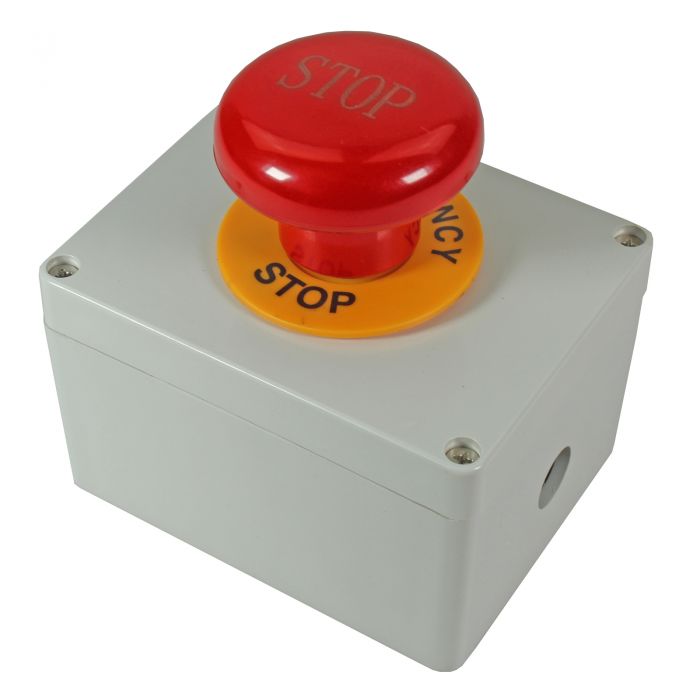The image depicts a close-up view of a small, rectangular gray box designed for emergency use. Prominently featured in the center is a large, red, mushroom-shaped button with the word "STOP" inscribed in cream-colored letters. Surrounding the base of this red button is a yellow disc with black lettering that reads "EMERGENCY STOP." On the right-hand side of the box, there is a round hole, slightly above the base, likely meant for wire installation. The box's lid is secured by four silver Phillips head screws, one in each corner. This emergency stop button is typically used in elevator firefighting systems or similar emergency scenarios to immediately halt operations when pressed.